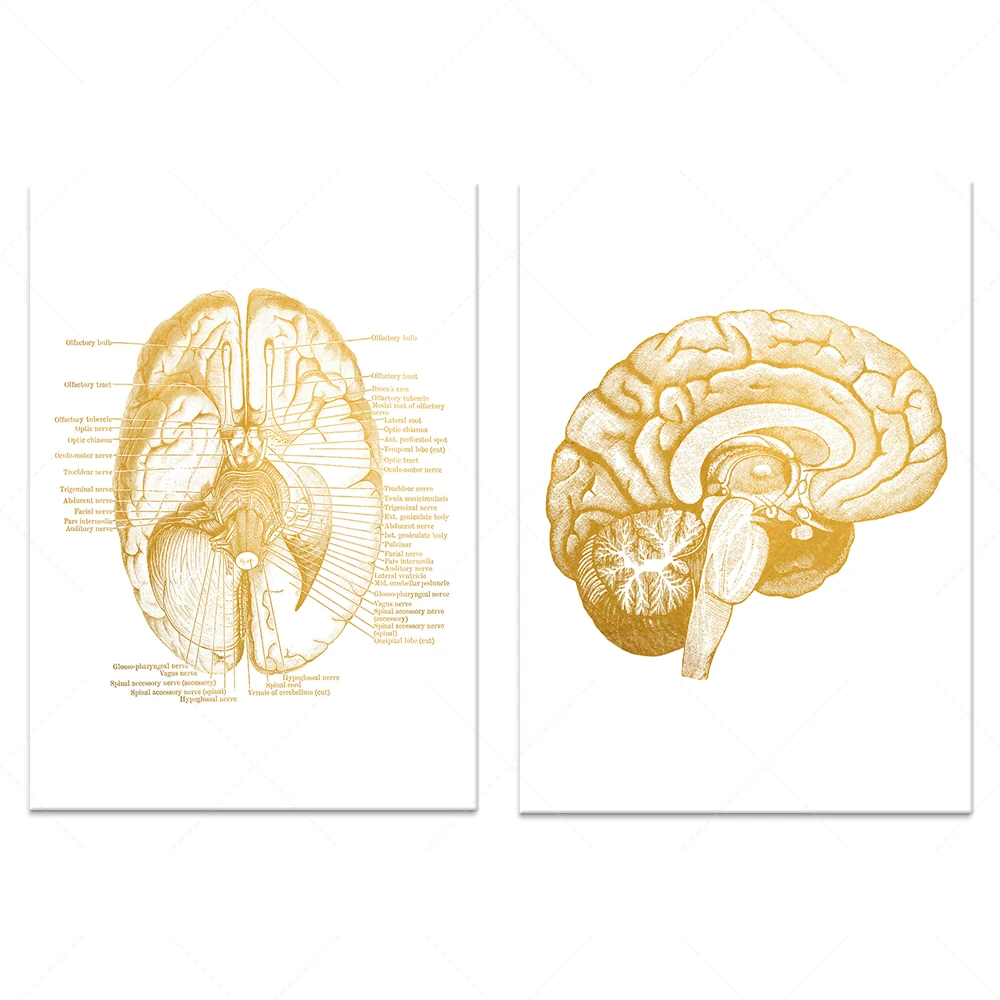The image features two detailed drawings of the human brain, each emphasizing different perspectives. On the left, there is a top-down view of the brain, displaying the two hemispheres and the central mechanisms. Each part of the brain in this view is meticulously labeled with text and arrows, though the writing is too small to read clearly. The diagram uses orangey-white lines and darker orange text to highlight the brain's intricate structure. On the right, there is a side view of the brain, showcasing a cross-section that reveals its internal components. This illustration is similarly colored in shades of orange and tan and is set against a white background. Both images together provide a comprehensive comparison of the brain's anatomy from different angles.